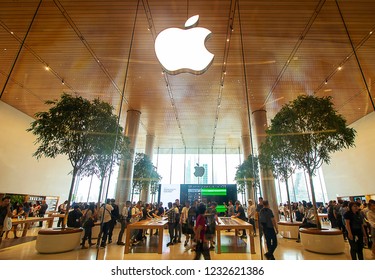This image depicts a bustling Apple Store, likely sourced from Shutterstock. The interior features tan walls flanking either side, with a row of tall windows along the back, allowing natural sunlight to flood the space. The ceiling boasts a vaulted design made of wood, prominently displaying a large Apple logo at the peak. On both the left and right sides of the room, neatly arranged in white pots, stand lush green trees. 

A central aisle is lined with sleek tables, showcasing various Apple products that attract numerous customers scattered throughout the room. The store's floor is a warm brown hue, complementing the overall aesthetic. Crowning the back center of the space is a large monitor with a black display and a green bar at the top, adding a modern touch to the environment. 

The content at the bottom of the image credits Shutterstock, with the code “1232621386,” indicating the photo's origin from this stock photography website.